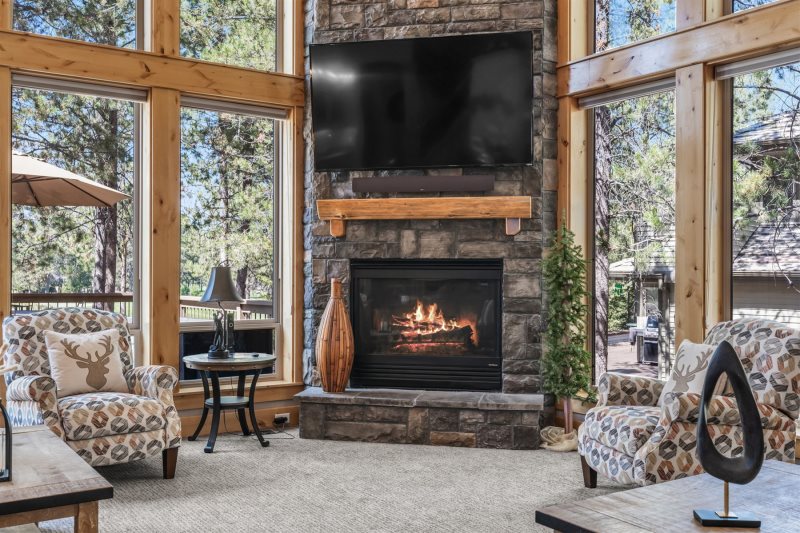The photograph depicts an expansive open living room, featuring large, uninterrupted windows framed by substantial wooden planks that allow a generous view of the verdant outdoors. The windows, set both to the left and right sides of the room, stretch from a wooden base upwards, enveloping the room in natural light. Outside, we see a wooden deck, a veranda umbrella, numerous lush green trees, and on the right side, a small barn with a grill and various objects placed beside it.

Dominating the center of the room is a striking fireplace, constructed from a mix of brown and gray splotched bricks, exuding a rustic charm. The fireplace is ablaze, with flames visible through a black mesh screen. Above the fireplace sits an LCD TV, also framed in black, perched on a wooden stand. Flanking the fireplace, to the left, is a brass vase with a lid on a lower mantel. Adjacent to the vase stands a nightstand featuring a beige lamp and a small figurine.

Further left, a comfortable armchair decorated with a circular pattern adds a cozy touch, complemented by a beige pillow with an orange silhouette of a deer's head. Near this area is a wooden table partially cut off in the image, topped with a black object. A matching chair and table with a similar black object are situated on the right side of the room, creating symmetry.

The room is anchored by a beige carpet, enhancing the warmth and inviting feel of the space. The overall decor combines elements of unfinished wood and modern functionality, with a charming blend of rustic and contemporary aesthetics. The photograph captures the scene during daylight hours, providing a bright and inviting ambiance.